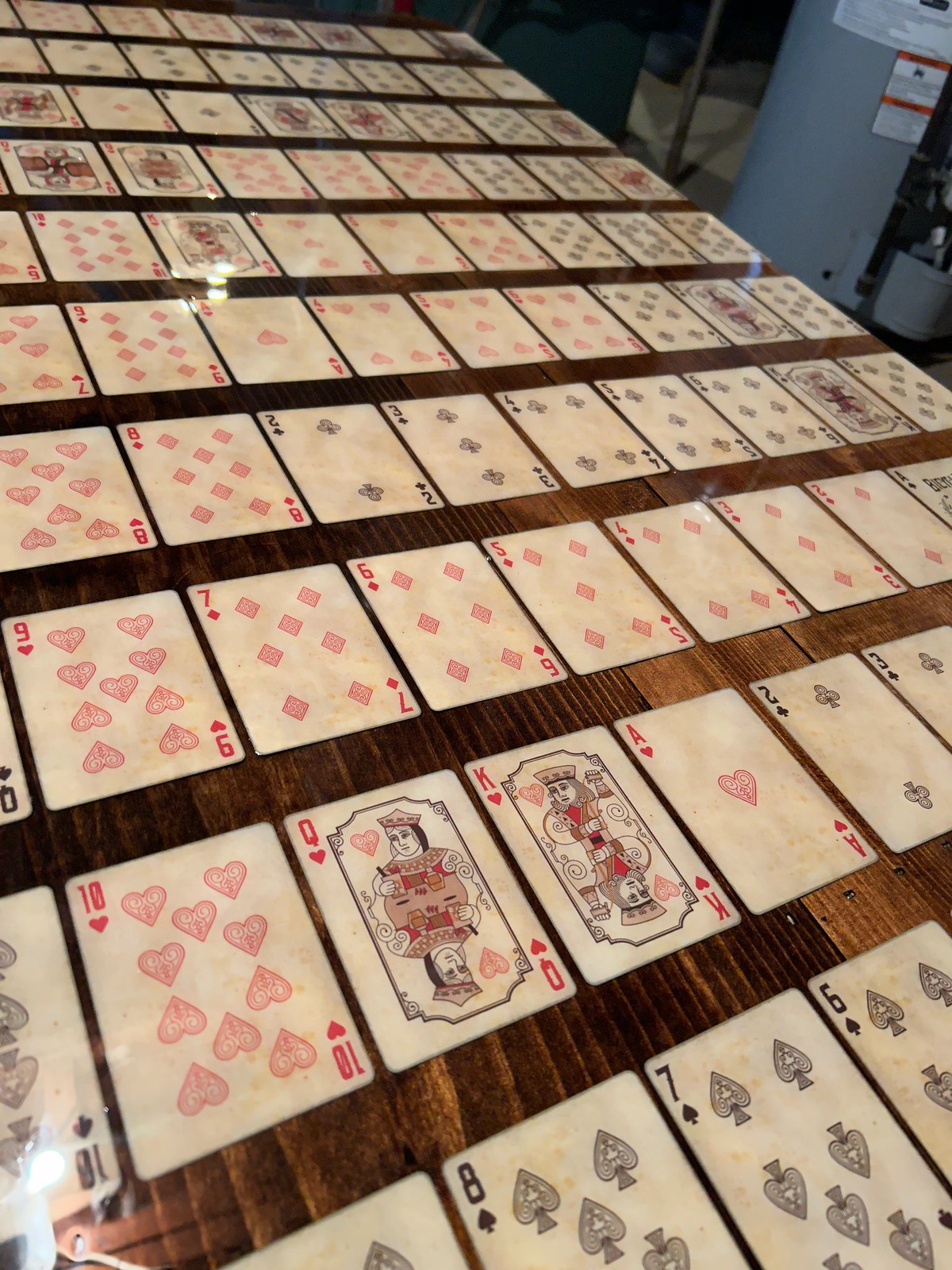The indoor color photograph showcases a unique wooden table viewed from above, extending diagonally from the upper left to the lower right and lower left corners of the image. The tabletop is made of natural, stark wood, laminated or shellacked over to embed a deck of playing cards. These cards are meticulously arranged in neat rows and columns, perfectly faced up. The rows are evenly spaced approximately an inch apart, allowing the underlying wood to be visible, while the columns have a narrower separation of about a quarter of an inch. The cards are not organized by number, suit, or face value, creating a random yet visually appealing mosaic. Notable cards, like the Ten of Hearts, Queen of Hearts, King of Hearts, and Ace, are discernible among the array, particularly near the center and lower left of the table. In the upper right corner of the image, the base of a gray water heater is partially visible, adding a touch of industrial contrast to the scene. A slight light glare can be observed in the upper left corner, indicating illumination from a light source above.